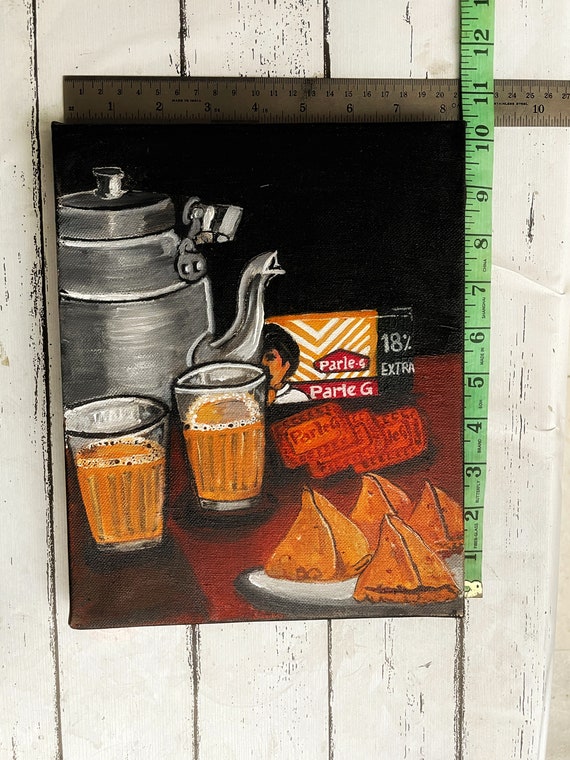The painting, hung on a white tiled or wooden paneled wall, depicts a contemporary and modern still life scene. Measuring approximately 11 x 8 inches, as indicated by a ruler placed horizontally on the top edge and a tape measure running vertically along the side, the detailed artwork captures various items arranged on a red table. Central to the painting is a large silver teapot accompanied by two glasses filled with a yellow or orange liquid, presumably tea. Next to the teapot, a box of Parle-G biscuits is prominently displayed, marked with "18% extra." In front of the box are what seem to be fortune cookies and possibly some orange tea packets. The background of the painting is dark, providing contrast to the colorful objects in the foreground. Overall, the painting's vibrant and meticulously crafted elements create a visually engaging composition.